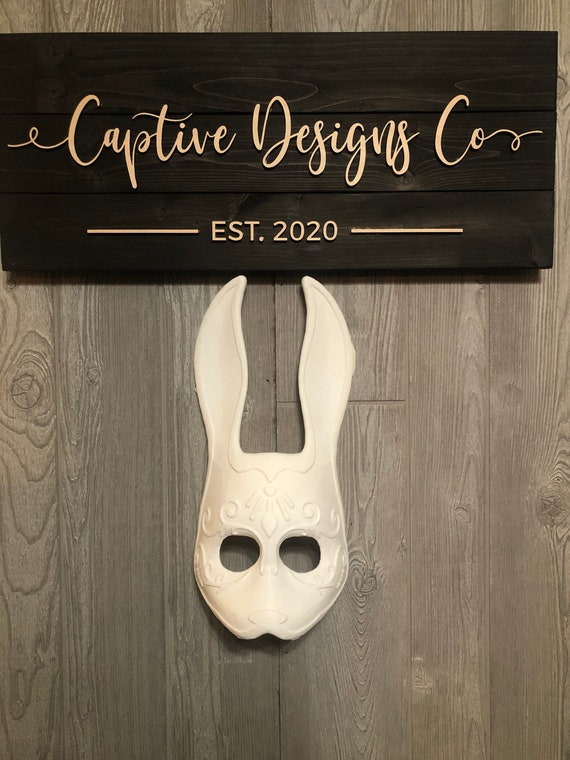The image captures a detailed photograph of an intricately designed white face mask resembling a bunny or rabbit, prominently placed at the center against a wooden background. The mask features large, vertical rabbit ears and two rounded eye holes, extending down to cover the nose but leaving the chin area exposed. The wooden backdrop is grey with a grainy texture, possibly machine-made as the planks appear seamlessly connected. Affixed towards the top of the background is a dark wooden sign comprised of three horizontal slats. In a beige cursive script, the sign reads “Captive Designs Co.”, with lines flanking the text on either end, followed by “EST 2020” beneath. The overall composition reflects a blend of rustic and sophisticated elements, highlighting the mask as a stylish fashion accessory within an indoor setting.